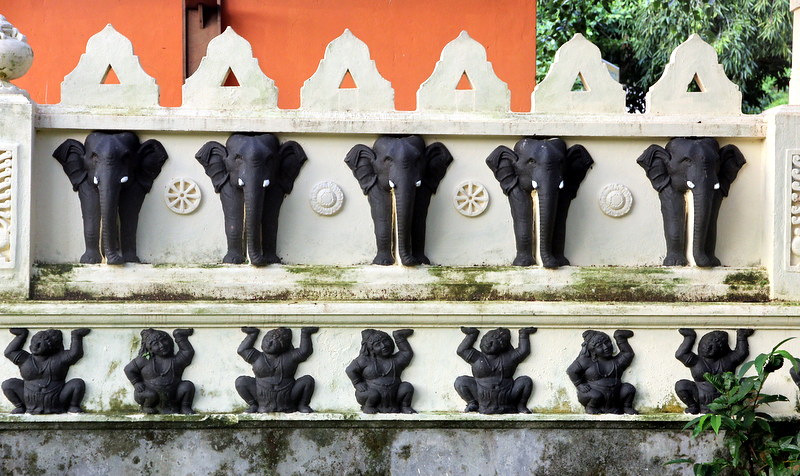The image is an outdoor photograph of a decorative wall or fence set against the backdrop of an orange building and lush greenery. The wall features white ceramic or concrete shelves holding intricate statues. The top shelf displays five black elephant statuettes with light blue or white tusks, positioned side by side with circular designs in between, resembling wheels and flowers. Below them, there is a row of seven black figurines, possibly representing female Buddhas or goddesses, each crouching with varied arm positions—either raising one hand or both, appearing to support the shelf above. The wall itself is mossy, adding a layer of green texture to the scene. At the top of the wall, six decorative, triangular shapes with cut-out centers line the structure, completing the ornate display. The two wooden pillars seen to the sides are partially cut out of the image. Dense greenery from a nearby tree fills the top right corner, adding to the serene and natural outdoor setting.